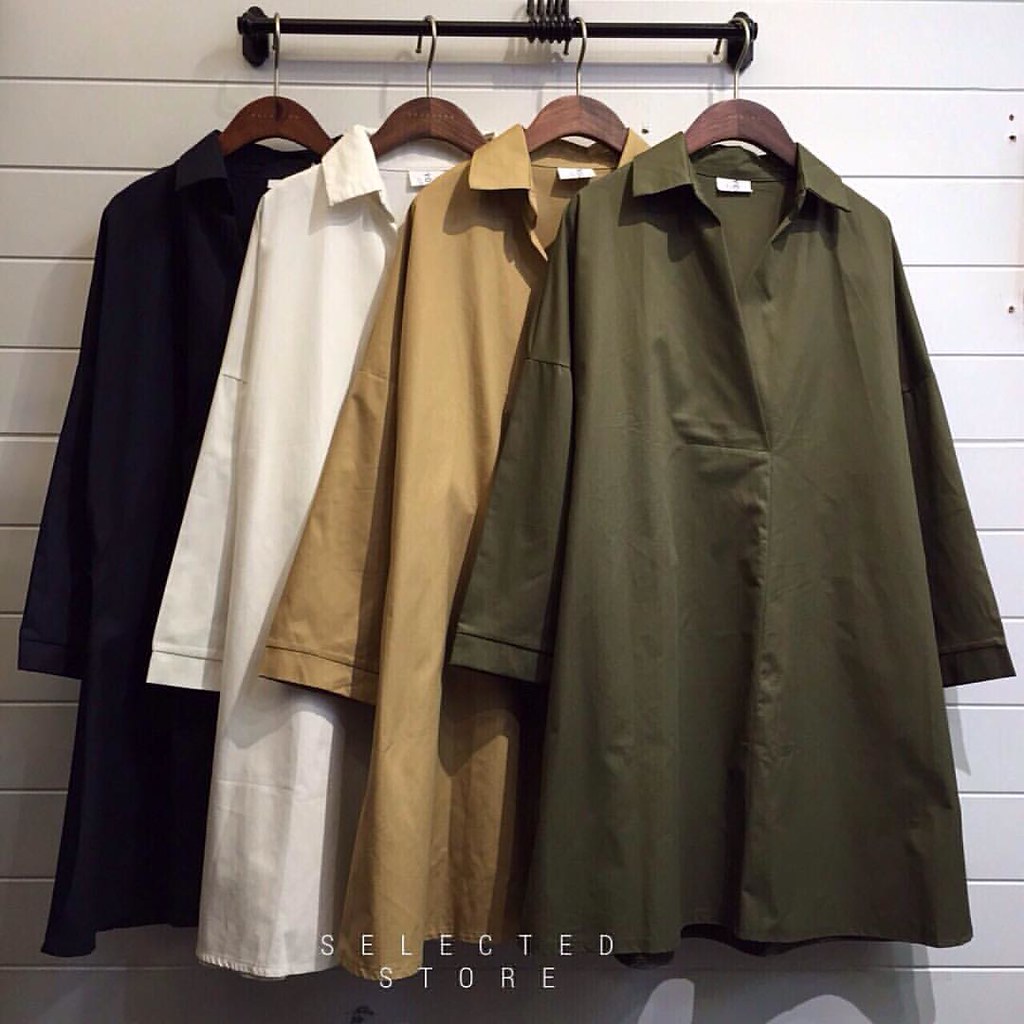The image is a color photograph, seemingly an advertisement for a clothing store, as indicated by the text "SELECTED" on one line and "STORE" on the second line at the bottom in white letters. The scene captures four women's tops or smocks, all of the same loose-fitting style and size, hanging on a black horizontal rail affixed to a white, horizontally paneled wall. Each garment is suspended from a dark brown wooden hanger with a metal, question mark-shaped hook. Positioned from right to left in a staggered, slightly overlapping arrangement, the tops are presented in the following colors: olive green, mustard yellow (or possibly light brown), white (which might also be extremely light pink), and a very dark color that could be black or navy due to the image's subtle lighting variations. The tops feature an open front similar to the length of a half-zip hoodie and various seams down the sleeves and towards the hand area, suggesting a functional design. The overall lighting of the image illuminates the top right corner more brightly while leaving the rest in softer light.